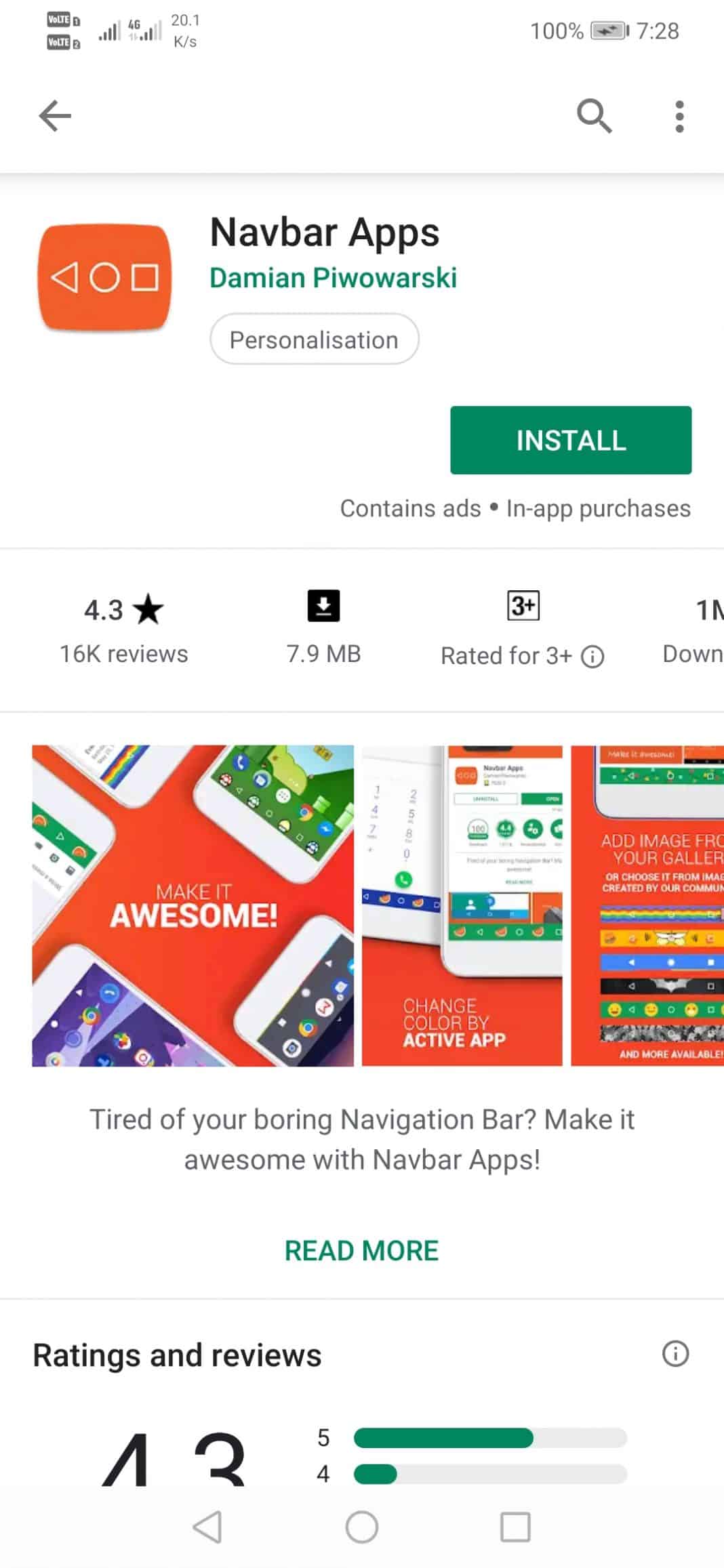Screenshot of the NAVBAR Apps page on the Google Play Store: 

The upper left of the screenshot features an orange icon with outwardly curved sides resembling a rectangle. The icon's center contains white outlines of a sideways triangle, a circle, and a square. To the right of this icon, the app's name, "NAVBAR Apps," is displayed in bold black text. Below the app name, the developer's name, "Damien Piwowarski," is written, with "Damien" in green and the last name in a mix of uppercase and lowercase letters.

Further down, there is an oval icon with a light gray border and the word "Personalization" written in gray lettering, indicating the app category. Toward the bottom right, a green rectangle stands out with "INSTALL" written in bold, capitalized white letters at its center. Below this button, small gray text notes that the app "Contains ads" and "In-app purchases," separated by a bullet point.

A faint gray line acts as a divider. Below this line, the app's rating is prominently displayed: "4.3" in dark gray or black, followed by a filled star. Below the rating, "16K Reviews" is written in gray text. To the right, a black square icon with a downward arrow and an underline indicates the app's size, "7.9 MB." Further to the right, the content rating is shown with a black square outline, featuring the number "3" and an additional symbol, along with the text "Rated for 3+" and a gray-bordered circle with a lowercase "i" inside.

The detailed layout provides all essential information about the NAVBAR Apps, making it easy for potential users to assess and download the app.